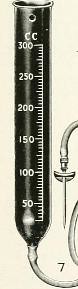The illustration is a narrow vertical strip on an off-white background, resembling the texture of parchment or old paper. Centrally featured is a black-colored test tube. The test tube is distinctly depicted with an open top and a small hole just below the rim. The upper part of the test tube is labeled with "CC" in white font, followed by "300". A horizontal line extends from the "300" marking towards the left margin, continuing vertically down the length of the illustration. This vertical line is segmented by multiple dashed lines, each marked with descending numerical labels: 250, 200, 150, and 100. The numbers are written in a downward sequence along the left side of the vertical line. The entire image appears to be either ink-drawn or printed on the paper.

Additionally, a narrow tube extends from the bottom of the test tube, curling gracefully out of the frame to the right and turning upwards, with its curly end reaching around the 150 mark on the test tube. The meticulous illustration, with its precise dashes and labeled measurements, exudes a scientific feel, emphasizing the clarity and accuracy of old-school scientific diagrams.